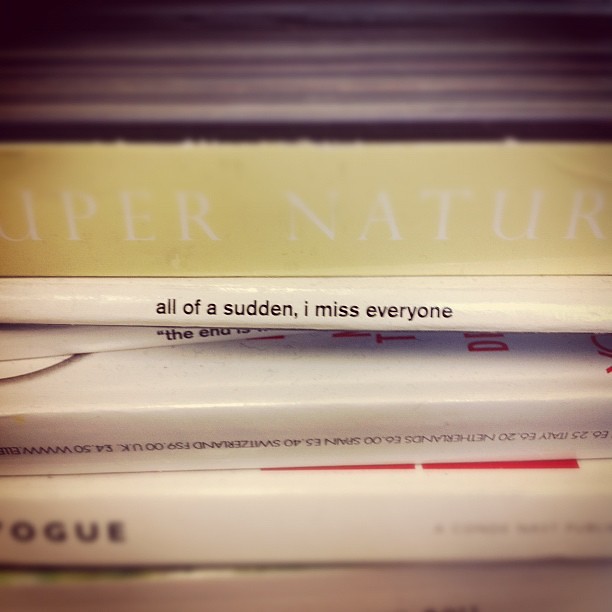The image captures a stack of six books, viewed from the perspective of their spines. The top book is thick with a yellow spine; the title "Super Nature" is partially visible, with only "uper Nature" readable due to the cut-off. The second book is thin, white, and displays the title "All of a Sudden I Miss Everyone" in black font. The third, also thin and white, has the phrase "The End Is" legible, but the rest is obscured as it is pushed into the stack. Below it, a fourth book has its title upside down, showing a string of characters and numbers like "E6, 25 Italy, E6, 20 Netherlands, E6, 00 Spain, E5, 40 Switzerland, FS, 9, 00 UK". The fifth book is a thicker white one with the partial title "O-G-U-E," suggesting it might be "Vogue" but is cut off on the left side. The composition of the books and their varied spine orientations create an intriguing, somewhat chaotic visual, emphasizing the randomness and diversity of the collection.